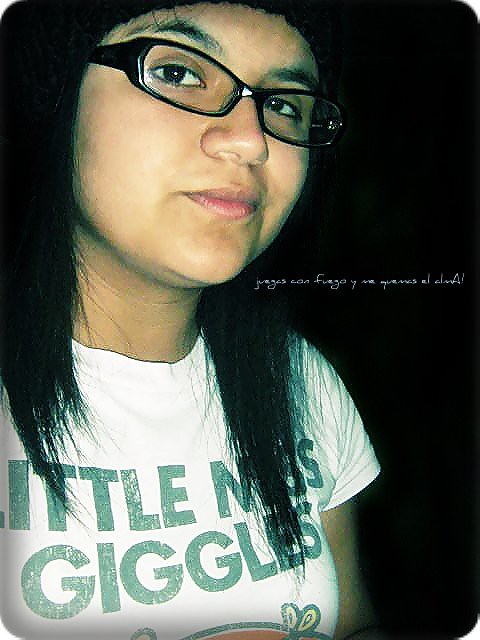The image features a teenage girl with long, straight black hair, partially covered by a beanie, which falls over both shoulders. She has distinct dark eyebrows, dark eyes, and is wearing thick, dark-framed glasses. She is dressed in a white t-shirt that reads "Little Miss Giggles" in blue text, with part of a cartoon character partially visible. The character appears to be an orange figure with arms and legs. The background is solid black, and the bright flash of the camera highlights her features, suggesting the photograph was taken in a dimly lit environment. The girl is looking towards the camera with a neutral or slightly smirking expression. There is a white watermark in the middle right portion of the image, written in Spanish, in a small, cursive font which is difficult to read. The photograph has a chill and casual aura, capturing an unguarded moment.